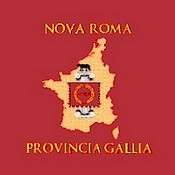This small, square image features a dominant red background with the words "Nova Roma" at the top and "Provincia Gallia" at the bottom in gold lettering. The central focus of the image is the yellow silhouette of a province or region with irregular edges. Centrally placed within this yellow outline is a smaller red square, containing a gold laurel wreath split into two halves. Above and below this smaller red square, there are additional elements that resemble a black and white Pac-Man viewed head-on. The overall design of the image appears somewhat blurry, yet the distinctive font and decorative elements suggest an elegant and formal representation of the region it depicts.